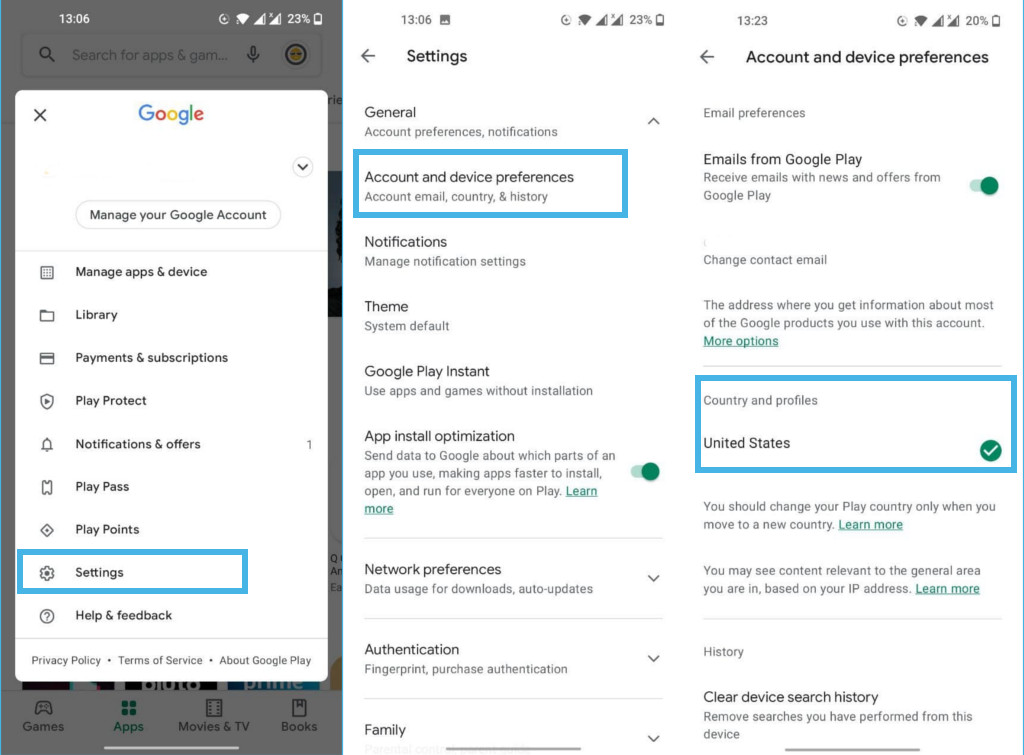This image features a composite of three different mobile screenshots, each capturing various settings menus within a Google Play application. 

The first screenshot, taken at 13:06, displays a white menu box listing several options: "Manage apps and device," "Library," "Payments and subscriptions," "Play Protect," "Notifications and others," "Play Pass," "Play Points," "Settings," "Help & feedback." The "Settings" option is highlighted with a blue rectangle, indicating selection.

The second screenshot, also taken at 13:06, shows the "Settings" menu in greater detail. The options here include: "General," "Account and device preferences" (highlighted in a blue rectangle), "Notifications," "Theme," "Google Play Instant," "App install optimization" (with a toggled-on green slider), "For preferences," "Authentication," and "Family."

The third screenshot, taken at 13:23, reveals the "Account and device preferences" section. At the top, the text "Account and device preferences" is displayed in black. Below this, there are options such as "Email preferences," where "Email from Google Play" is toggled on with a green slider, and "Change contact email." Additionally, there is a blue rectangle with a green check mark next to "United States" under the "Country and profiles" section. At the very bottom, an option to "Clear device search history" is present.